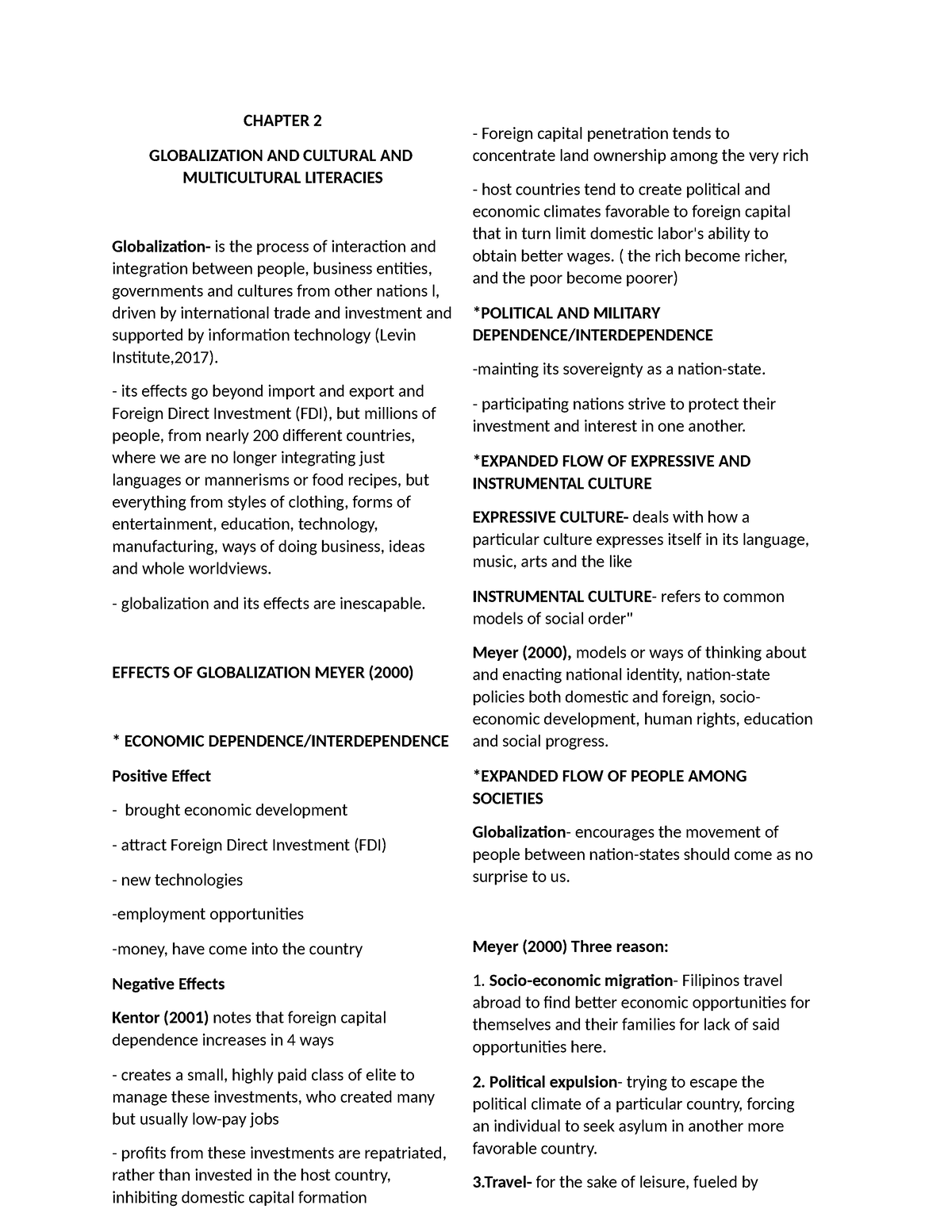This image features a detailed text layout, divided into two columns, all set against a white background with black text for clear readability.

The left-hand column begins with the heading "Chapter 2, Globalization and Cultural and Multicultural Literacies." It defines globalization as the process of interaction and integration among people, businesses, governments, and cultures from different nations. This complex phenomenon is primarily driven by international trade and investment, supported by advancements in information technology. The text emphasizes that globalization's impact stretches beyond just import and export or foreign direct investment. It involves millions of people from nearly 200 countries, where integration transcends languages, mannerisms, and food recipes to include elements such as clothing styles, entertainment forms, education, technology, manufacturing processes, business practices, ideas, and entire worldviews. This column also discusses the effects of globalization, citing Meijer (2000), and touches on economic dependence and interdependence, listing both positive and negative results.

The right-hand column continues exploring these themes, with headings such as "Political and Military Dependence" and "Interdependence" followed by "Expanded Flow of Expressive and Instrumental Culture." This section explains the terms 'expressive culture' and 'instrumental culture.' Furthermore, it discusses the "Expanded Flow of People Among Societies," noting how globalization fosters the movement of people between nations. This part also refers to Meijer (2000), highlighting three reasons for such movements: socioeconomic migration, political expulsion, and travel.

This comprehensive text sheds light on the multifaceted nature of globalization and its wide-reaching effects on various aspects of global society.